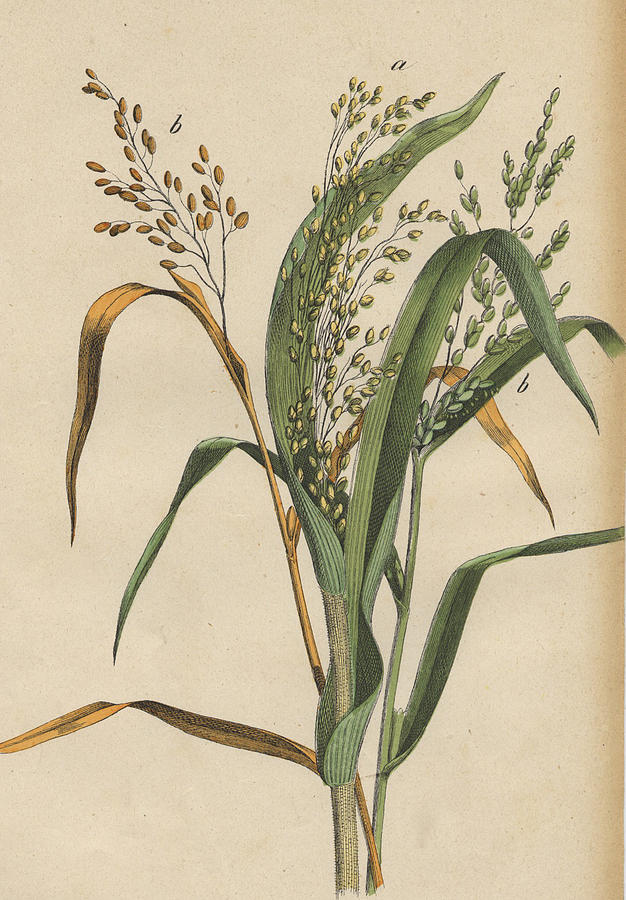The image depicts a pen and ink artwork with muted colors on a light brown, almost parchment-like background that transitions to a slightly darker shade on the right side. The artwork measures approximately six inches tall by four inches wide. At its center stands a plant with a thick main stalk, reminiscent of a corn stalk but without any flowers. Instead, it features small sections that might represent seeds. The primary stalk is green, extending leaves that curl downwards under their own weight. Behind it, a thinner goldenrod-yellow stalk adds contrast. From these stalks, thin tendrils emerge, each adorned with small, rounded grains or seeds that shift in color—from green near the green stalk to golden as they approach the goldenrod stalk. The delicate interplay of green and golden hues and the meticulous detailing evokes a sense of nature's intricate beauty captured in a subdued palette.